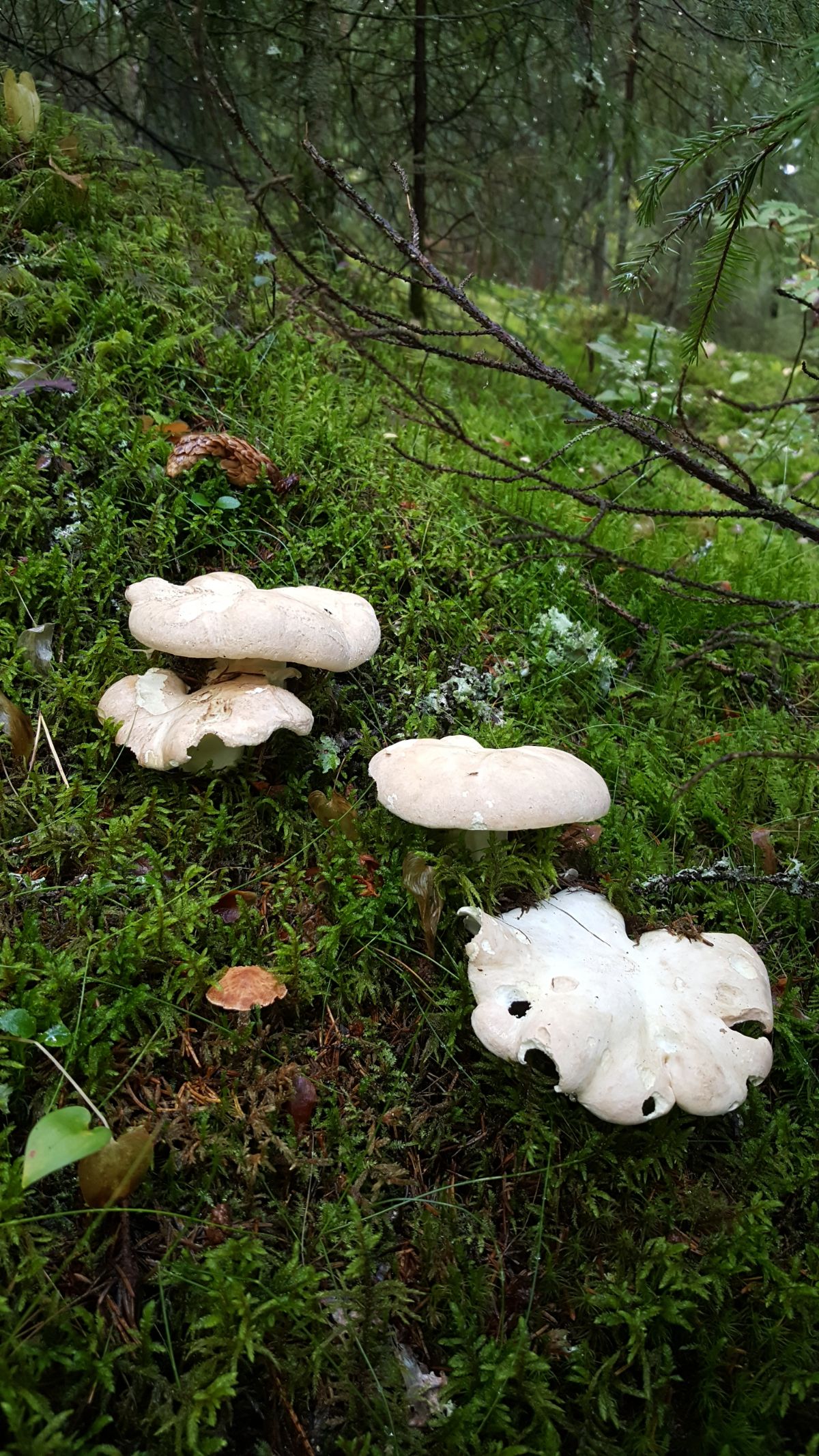In this photograph, we see a detailed forest scene focusing on a cluster of diverse mushrooms on the forest floor. Dominating the foreground are four larger off-white mushrooms, likely resembling oyster mushrooms in shape, though they are likely of a different variety. These mushrooms display a creamy, off-white color with some irregularities and waviness to their edges, suggesting that some small creature may have nibbled on them. Nestled among them is a smaller brownish mushroom to the bottom left. 

The forest floor is lush with short grass, moss, and patches of lichen, hinting at a damp, possibly recently rained-upon terrain. Toward the top of the photograph, several tree branches and a stand of trees stretch into view, framing the scene and providing context to the mushrooms' woodland habitat. Additionally, the ground slopes gently downward, indicating a hillside, with subtle details such as pine leaves, small sticks, and even an acorn peeking through the greenery. In the background, a faint silhouette of a house can be discerned, adding depth and a sense of place to the natural tableau. Overall, the image captures a rich, verdant slice of forest life, alive with detail and texture.